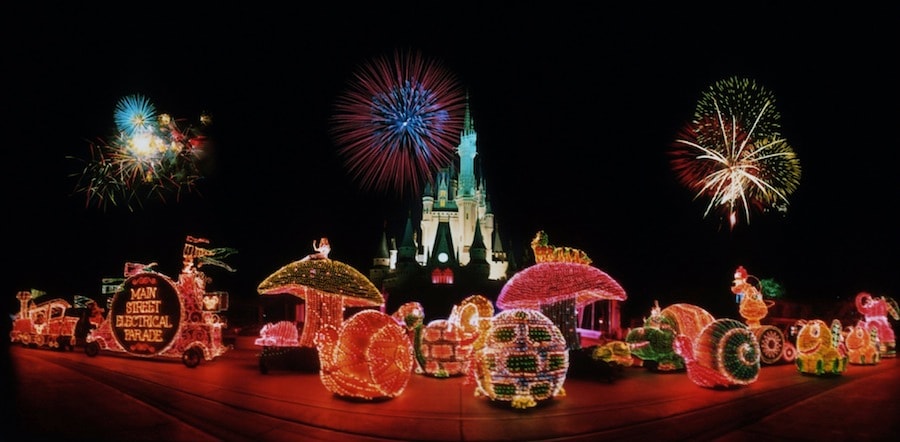The image captures a nighttime scene at Disneyland, with the iconic Disney Castle illuminated in blue and white, taking center stage in the background. Fireworks explode in the sky, with at least three bursts lighting up the dark, almost jet-black night. In the foreground, a stage is set up with various whimsical, illuminated decorations. Large, glowing snails and mushrooms dominate the center, accompanied by other light-up figures such as turtles and diverse animated characters. These figures and decorations stretch from the bottom left to the bottom right, casting a bright, colorful array of darkish oranges, yellows, bright blues, greens, reds, pinks, and bluish purples across the scene. The ground beneath these displays is reflective, enhancing the vibrant and festive atmosphere. The overall setting suggests a lively event or showcase, possibly for entertainment or advertising purposes, reminiscent of Disneyland's magical and enchanting ambiance.